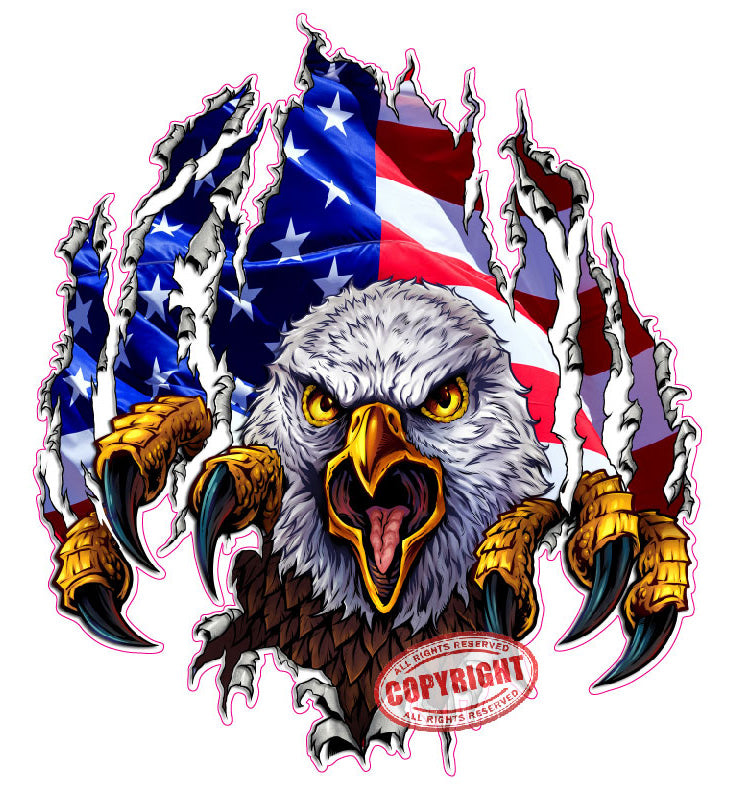The image depicts a dynamic graphic design intended for a shirt, set against a white background. At the center is a fiercely rendered illustration of a bald eagle with a white head, piercing yellow eyes, and a wide-open yellow beak revealing a reddish-pink tongue. The eagle appears to be lunging forward, its sharp, midnight-green claws tearing through the white backdrop. These rips, outlined in hot pink, expose a waving American flag behind the eagle. The flag features blue with white stars on the left and red and white stripes on the right, creating a striking contrast. Below the intricate visual, a white oval with a red outline displays the word "Copyright" in red letters, along with smaller text above and below that reads "All Rights Reserved." The design artistically combines elements of realism and illustration, emphasizing the bold imagery and patriotic theme.